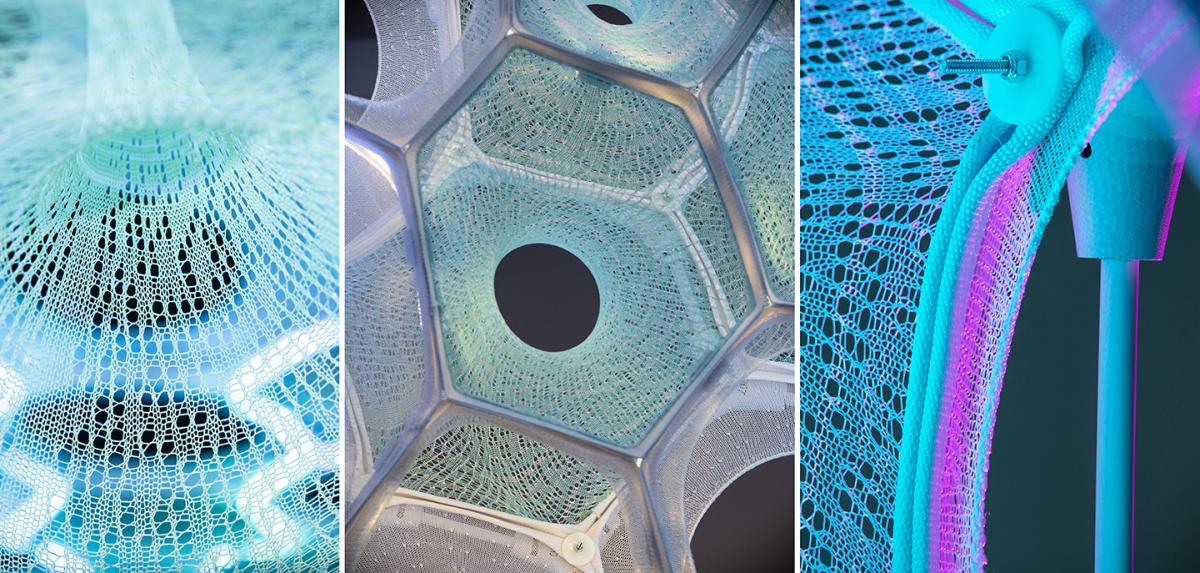The image showcases a series of three photographs side by side, each focusing on a brightly colored, porous mesh material. 

- **Left image:** A close-up view of a neon green and blue-white mesh that appears to be pulled upwards into a circular cone shape at the center.
  
- **Center image:** Features a hexagonal metallic grid where the mesh is stretched across the hexagons. The mesh displays a hole in its center, revealing a black void with a neon green hue, and the overall illumination gives the mesh a blue-white coloration. 

- **Right image:** Highlights the edge of a neon teal and hot pink mesh secured by a screw, washer, and nut, suggesting that the material is fastened to a frame. This image presents the material in a vibrant arrangement, stretching the fabric and giving off a honeycomb texture.

The collective imagery reveals a high detail of the mesh's structure, its usage, and how it interacts with lighting to produce varying neon shades.